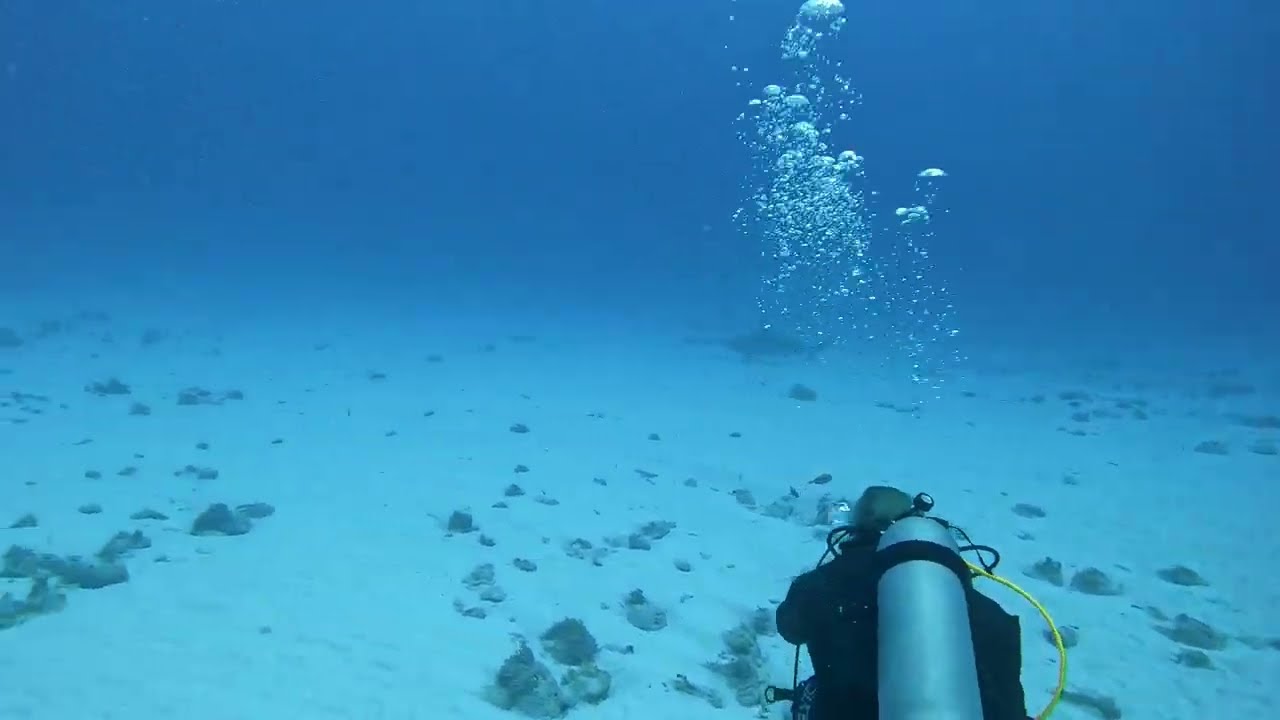An underwater photograph captures a diver in full black diving gear, positioned toward the center right of the frame near the sandy seafloor. The diver has a silver air tank attached to their back, connected to them via a yellow tube. A series of bubbles, prominently featuring a large one at the top of the image, rise above the diver, hinting at a recent exhalation. The sandy terrain is dotted with rocks, some of which are covered in marine plant life. In the background, a blurry silhouette, possibly a shark, looms near the bottom, adding an element of mystery, though it could also be mistaken for a large flat rock or a turtle. The water is a clear, vibrant blue, though some image compression makes fine details slightly fuzzy. The overall scene is devoid of other fish, encapsulating a serene yet enigmatic underwater environment.